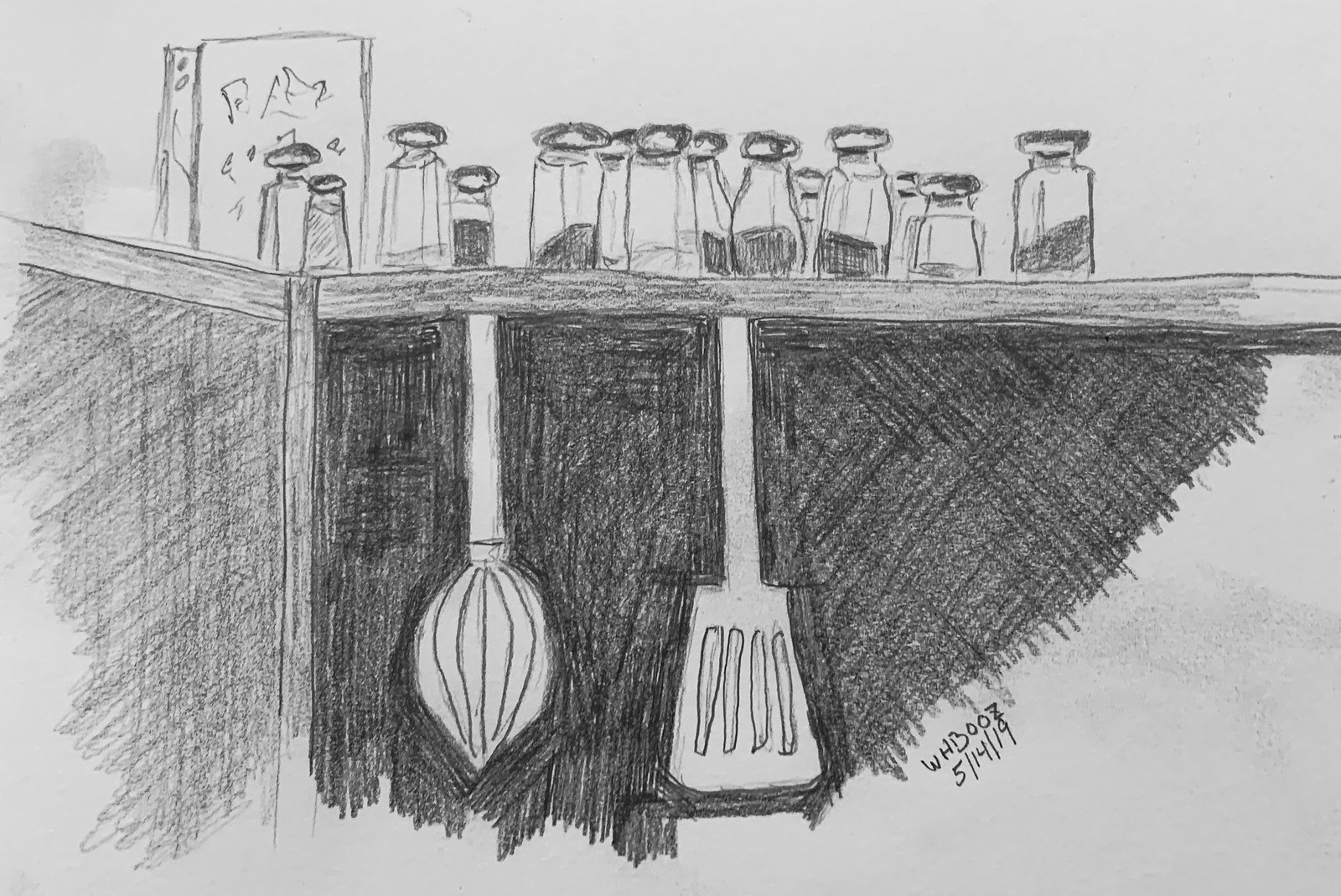A hand-drawn pencil sketch of a kitchen scene, showcasing a variety of utensils and kitchenware. Hanging from a countertop, a spatula and a whisk are prominently displayed. The background is intricately shaded with multiple black lines, giving it a textured, scribbled appearance. Below the utensils, the artist's signature "W.H. Booze" and the date "5-14-19" are visible. On the countertop, there are several small bottles, likely representing salt and pepper shakers, with distinct black and white contents. Additionally, a grater can be seen in the background, adding to the detailed depiction of the kitchen setting.